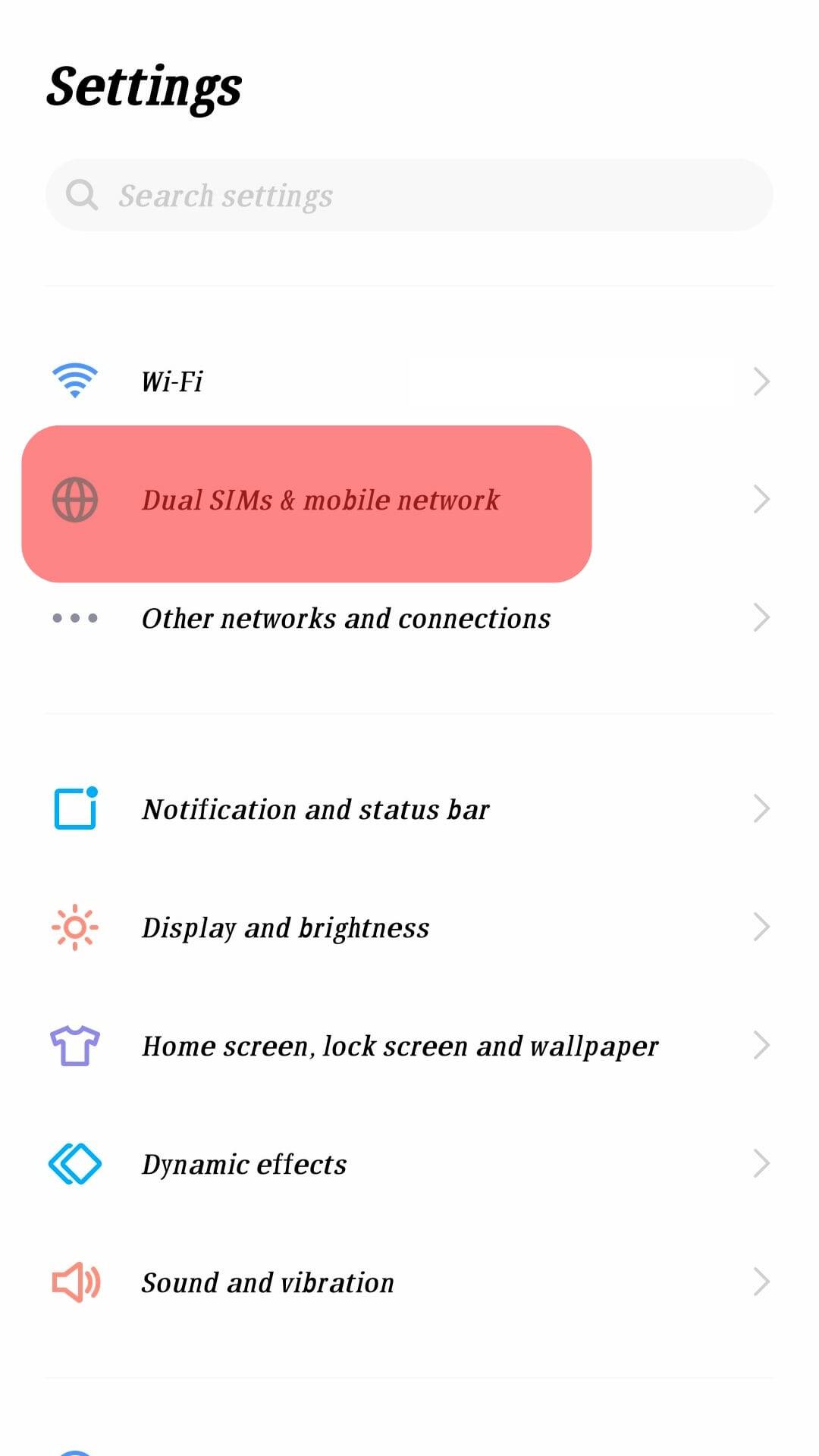This screenshot captures a settings page. The layout suggests it's intended for mobile, although there's no definitive indication it's a phone, as no icons, status bars, or navigation bars are visible at the bottom. The background is predominantly white, with black text.

In the top left corner, "Settings" is displayed in bold and italics. Below it, a gray search bar is labeled "Search settings." The first setting item features a blue Wi-Fi icon and an accompanying gray arrow. Moving down, "Dual SIMs and Mobile Network" is marked in red, represented by a globe icon with a curved rectangle overlay in a light red or dark pink hue. 

Further down the list, sub-sections include:
- "Other Networks and Connections" with descriptive dots 
- "Notification and Status Bar" with a blue square icon
- "Display and Brightness" featuring a red sun icon
- "Home Access, Lock Screens, and Wallpaper" indicated by a t-shirt edged in purple
- "Dynamic Effects," symbolized by two blue diamond shapes
- "Sounds and Vibrations," marked by a red sound icon

Each item is paired with a gray arrow on the right, implying they are expandable for more detailed settings.

Of peculiar note is a pink rectangle highlighting the "Dual SIMs and Mobile Network" section, which appears superimposed rather than naturally integrated, suggesting some form of manual emphasis or editing on the screenshot. This aspect stands out as an unusual modification to the standard settings interface.